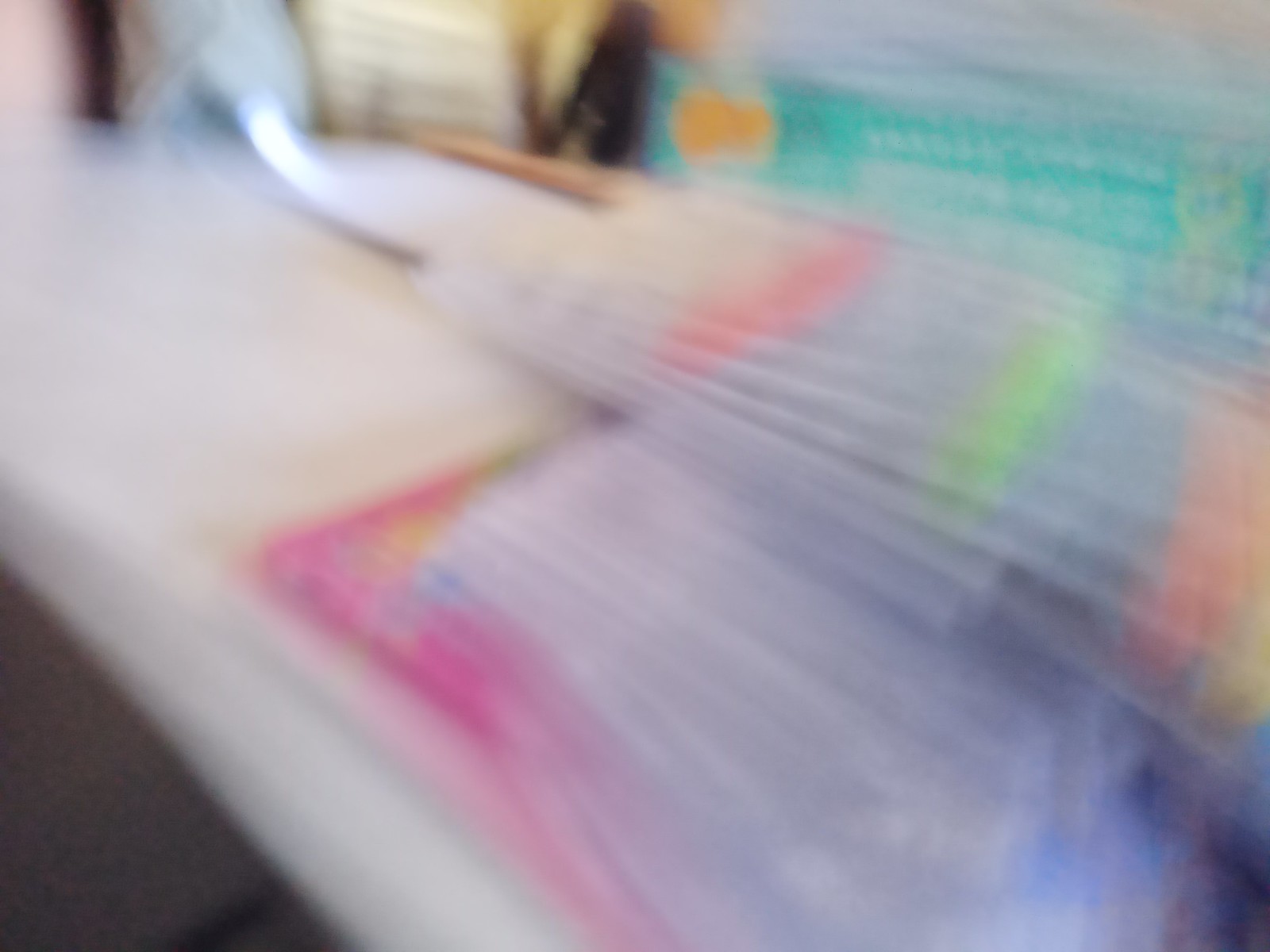The image is an extremely blurry photograph with a confusing array of elements, suggesting possible motion during capture. The central focus appears to be a series of stacked items, which could be newspapers, napkins, or possibly foreign currency, given their uniform appearance and repetitive stacking. These stacks feature a myriad of pastel colors, including pink, blue, purple, lime green, aqua, and orange. Among these stacked items, there is a noticeable purplish image with visible folds, emphasizing the stacked nature. In the top right corner, there's a green object that might be packaging, though its details remain unclear. The upper left corner features a metallic and shiny, hooked light source, which provides some illumination. The lower left-hand corner is dark and undefined. Overall, the image presents an array of blurred, pastel-colored objects stacked up on what seems to be a white counter, stretching diagonally from the bottom center to the upper left side of the photo.